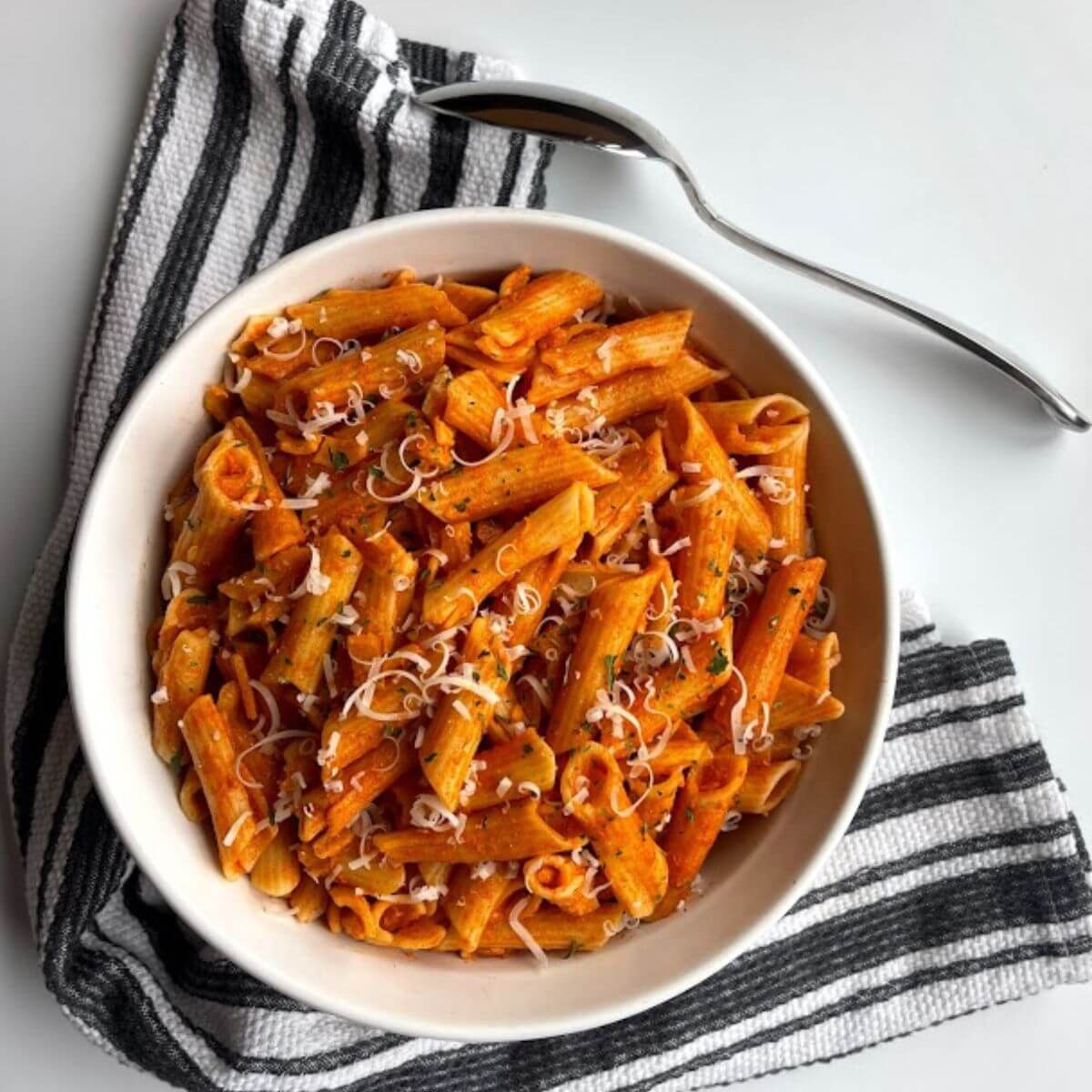In this detailed photograph, a ceramic bowl of Penne a la Vodka takes center stage, almost filled to the brim with cylindrical penne pasta coated in a rich tomato sauce. The pasta is attractively garnished with shavings of mozzarella cheese, a sprinkle of oregano, and a hint of coarse ground pepper, presenting a beautiful burnt orange color. The bowl rests on a distinct black and white striped kitchen towel that's arranged in an L shape atop a pristine white slate countertop. Adjacent to the bowl, a silver spoon lies sideways on the top right of the image, pointing towards the bowl, enhancing the overall aesthetic. The dish appears freshly baked, conveying a sense of warmth and home-cooked goodness.